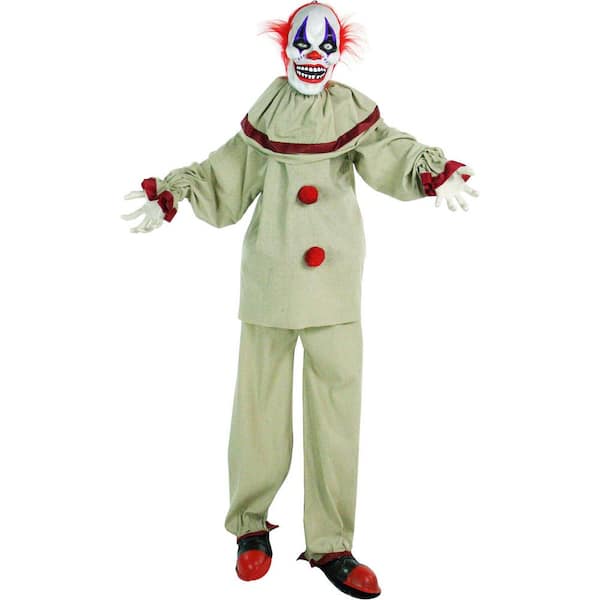An ominous figure stands before me—a photograph of a terrifying clown that exudes a chilling presence. This eerie clown is dressed in a pale tan or lightish olive outfit, accented with red outlines along the cuffs and the cowl of the garment. Prominently, two large red buttons adorn the front of the outfit, adding to its sinister look, along with a big white collar with a red stripe. Its footwear consists of striking red shoes with black stripes, completing the unsettling ensemble.

The face of the clown is a ghastly white, marked with grotesque makeup. Blue designs accentuate the area around its eyes, which are also highlighted by dark, menacing tattoos or makeup. The clown sports a red nose and jagged teeth framed by vivid red lipstick. Its hair is red but sparse, contributing to a balding appearance with tufts sticking out unsettlingly. The gloved hands are white, posed in a manner that suggests a claw-like readiness. Altogether, the figure seems poised to walk towards the viewer, amplifying its menacing and frightening aura.